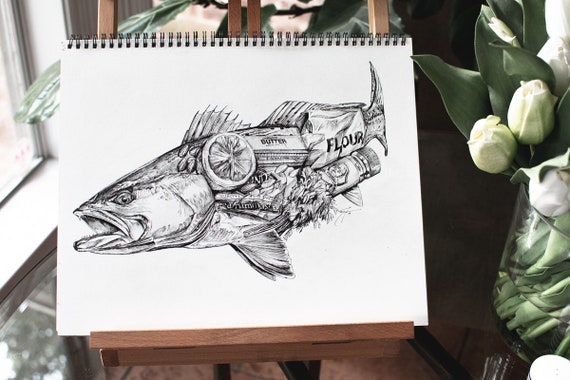The image depicts an intricate black-and-white ink drawing of a fish situated on a wooden easel, resting on a tabletop in a well-lit room. The fish is carefully crafted from various superimposed objects, including a lemon slice, a pat of butter labeled "butter," a bag labeled "flour," a piece of currency, a bottle, and some flowers, creating a textured collage within the fish's form. The background features a clean, white space, while to the right of the easel stands a clear vase filled with white tulips. To the left, light streams in through a partially visible window pane, illuminating the scene. The detailed drawing is housed in what appears to be an artist's sketchbook or journal. Despite the realistic depiction, subtle anomalies suggest that the image might have been generated by AI.